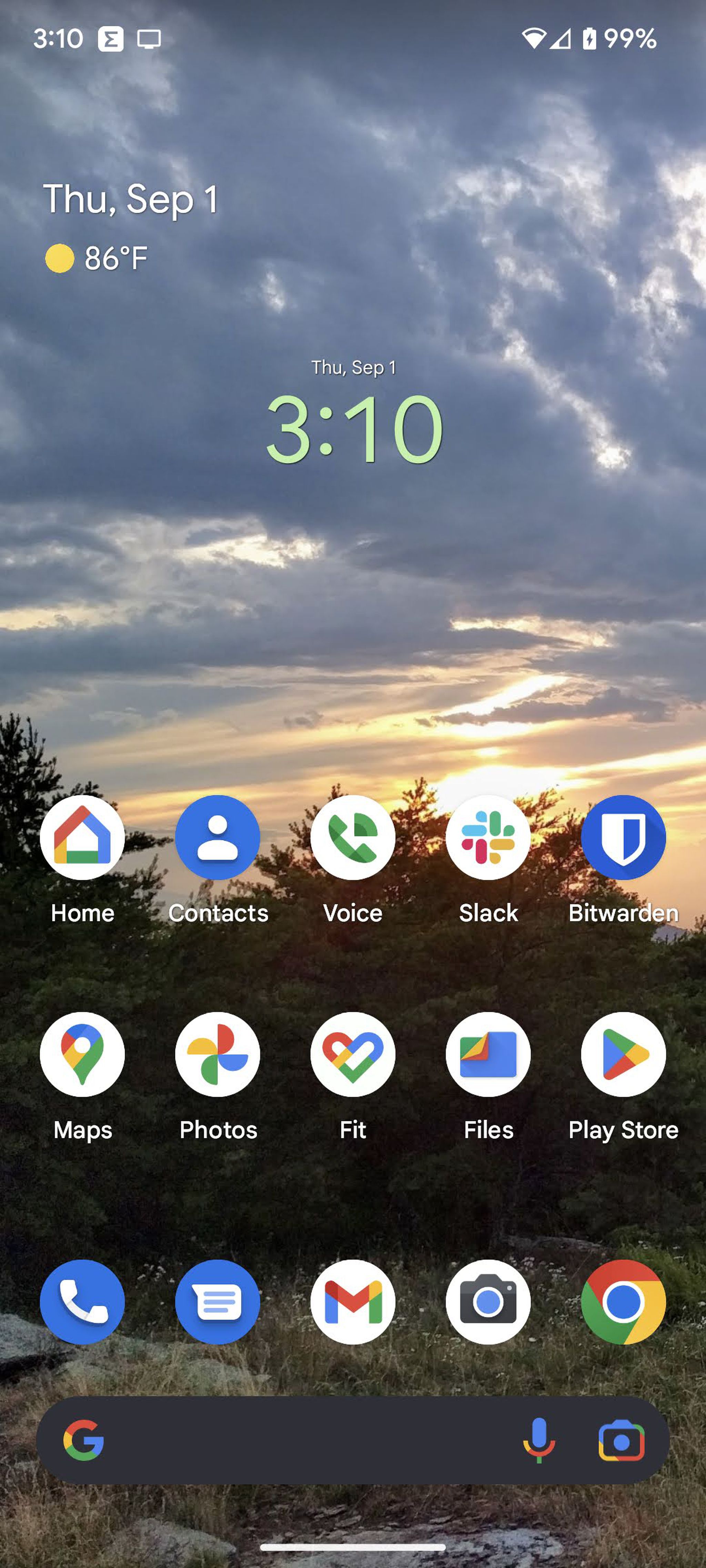Here is a cleaned-up and detailed descriptive caption for the image:

---

Screenshot of a smartphone display at 3:10 am/pm. The top right of the screen showcases a battery icon at 99% and an icon indicating low wireless signal. An inverted triangle icon to the left marks the availability of Wi-Fi. The background image displays a picturesque scene taken during sunrise or sunset, evidenced by the Sun near the horizon, casting a blend of bluish-red clouds across the sky. Below the sky, a dark tree canopy is silhouetted, with grass and stones faintly visible in the foreground.

At the top center of the screen, "THU SEP 1," denoting Thursday, September 1st, is displayed, with the time "3:10" shown prominently in large green letters. Repeating this information, the upper left part of the screen shows "THU, SEP 1" in white font below the time, followed by a yellow circle with "86°F" indicating the temperature.

The lower half of the screen is populated with 15 icons organized in rows. The first row reads: Home, Contacts, Voice, Slack, Bitwarden. The second row reads: Maps, Photos, Fit, Files, Play Store. The third row consists of icons: a Telephone (presumably calling), Messaging, Google Mail (Gmail), Camera, Google Chrome (illustrated by a circle with a blue dot in the center, red top, yellow lower right, and green lower left segments).

At the bottom, there is a gray Google search bar featuring the Google logo on the left and microphone and camera icons to the right. Finally, a horizontal white bar spans the very bottom of the screen, presumably to indicate the navigation handle for gesture control.